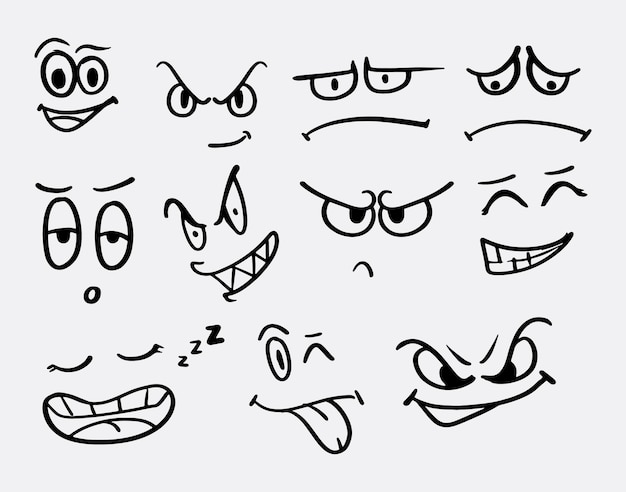This image features 11 cartoon-style, expressive faces arranged in three rows—four on the top row, four in the middle, and three on the bottom. The faces are hand-drawn in a comic book style, consisting solely of exaggerated eyes, eyebrows, and mouths, devoid of noses, ears, or head shapes. Each face vividly portrays a different emotion: the top row shows happiness, deviousness, disappointment, and sadness; the middle row displays mild surprise, anger, irritation/disappointment, and joy/amusement; and the bottom row includes tiredness/sleeping, silliness, and possibly another devious or mildly irritated expression. The drawings are monochromatic, rendered in black and gray.